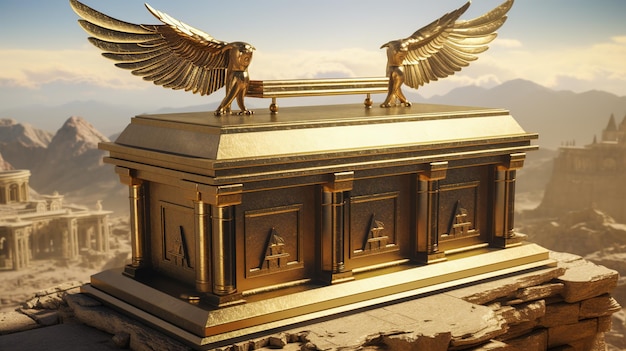The image is a detailed computerized render showcasing a gold sarcophagus set against a fantastical landscape with ancient architectural elements. The sarcophagus, gleaming solid gold, features a distinct design with triangular motifs on three side panels and a consistent pattern on the narrow end, flanked by two golden columns. Atop the sarcophagus, a handle-like structure sits between two intricate depictions of Horus, the Egyptian deity represented as a man with wings and a bird's head. The background reveals a vivid scene with a blue sky, scattered white clouds, and rugged dark mountains. Surrounding the central sarcophagus are large vulture-like birds with outspread wings, perched as though guarding it. Additional elements in the backdrop include tan-colored pillars with dark recesses and a light-hued castle-like structure nestled among the rocky cliffs. The interplay of light accentuates the golden surfaces and adds a mystical glow to the scene.